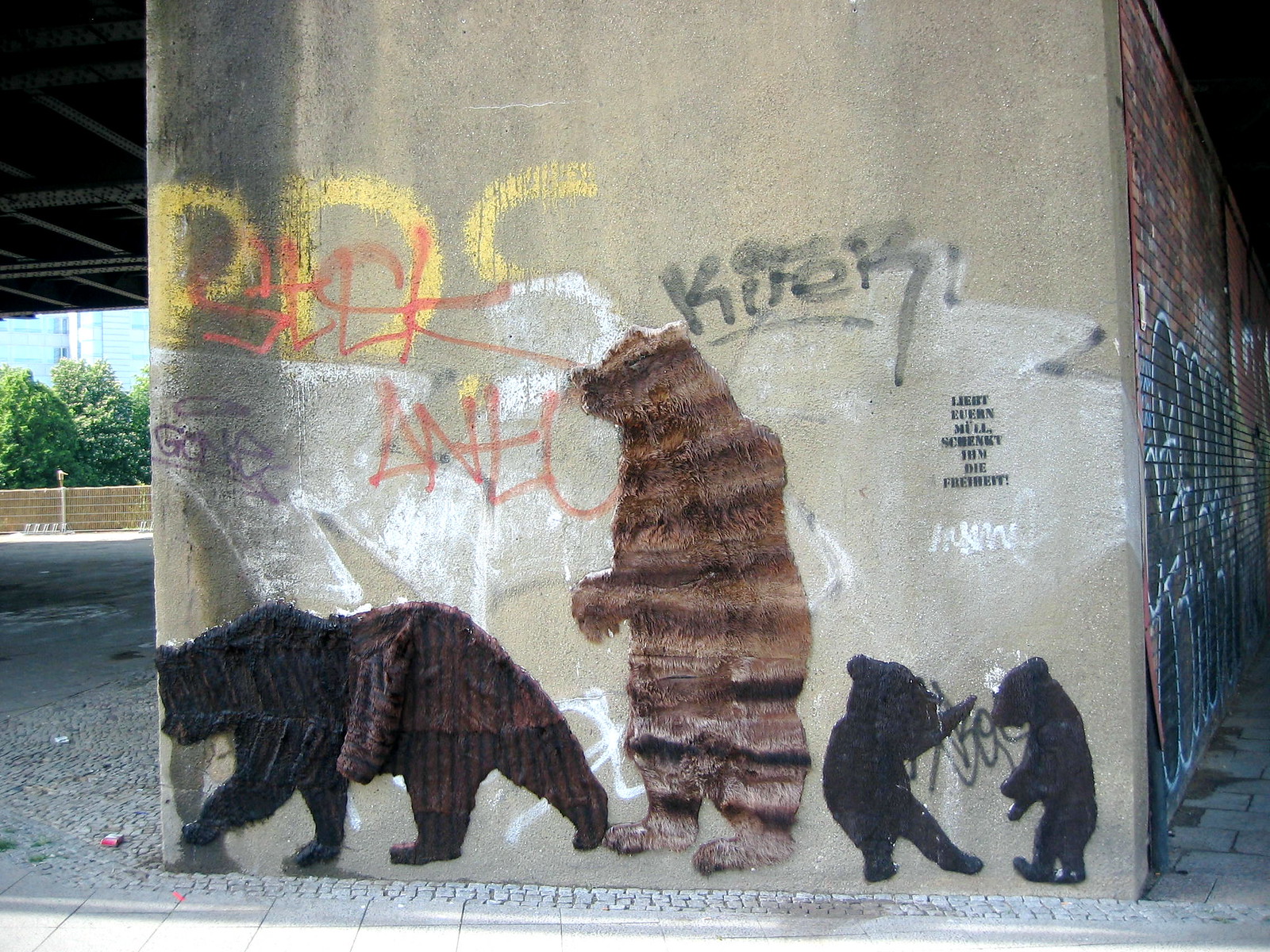In this vivid photograph, we see an industrial-looking setting, perhaps beneath an overpass, bridge, or in a parking lot. The main focus is on a large grey concrete wall, heavily adorned with graffiti and street art. Centered on this wall, there are four detailed depictions of bears crafted in different shades and positions. 

On the left side, a bear with a striking coat, half black and half dark brown, is depicted crawling or walking towards the left. In the middle, a lighter brown bear stands upright, seemingly gazing to the left. To the right, two playful cubs with black fur add a lively touch, interacting with each other.

Surrounding the bears, the wall is embellished with a variety of graffiti. Notable tags include "K.I.F.E.R." in black, "P.D.S." in yellow, "G.O.R.N.E." in purple with an oval halo, and other indistinct words and scribblings. A stenciled stamp-like font bearing miscellaneous words, including "IRJIT IRAN MUL SKORN KI DUM DAI FOR FRET," adds to the textural collage of graffiti.

The environment behind the wall reveals multiple details: a red brick wall on the right side, distant cityscape elements, hints of foliage and green trees, a streetlight, and some visible litter on the ground, underlining the urban atmosphere. The upper left corner of the image shows part of the roof of the industrial structure, painted dark black, completing the rugged look of this striking urban scene.